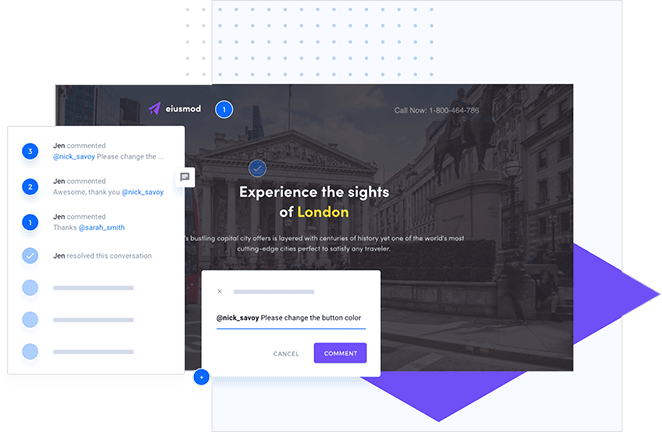This screenshot captures an overlapping array of objects within a landscape-oriented frame, seemingly related to a web development project. 

1. **Main Sections**:
   - **Left-Center and Bottom Area**: 
     There's a prominent white vertical box featuring a threaded history of comments. Each comment bubble is displayed in blue and numbered from 3 to 1, followed by lighter bubbles including a check mark and several blanks:
       - **Comment 3**: "Jen commented at Nick Savey, please change the..."
       - **Comment 2**: "Jen commented, awesome, thank you Nick Savey."
       - **Comment 1**: "Jen commented, thank you Sarah Smith."
       - **Check Mark**: "Jen resolved this conversation."
   - **Bottom-Center Area**: 
     Another white rectangular box contains the message "at Nick Savey please change the button color." Below this message, there are two buttons: a "Cancel" button and a purple "Comment" button.
   
2. **Background Elements**:
   - Behind the white boxes, a larger background image depicts a classical pillar-like building promoting an ad with text reading, "Experience the sights of London." 
   - The ad includes a logo, resembling a purple navigation arrow, and a "Call Now" button in white. The main text is in white with "London" highlighted in yellow.

Overall, the screenshot seems to depict a collaborative effort to edit a website, with various team members engaging in conversations about ongoing changes and enhancements.